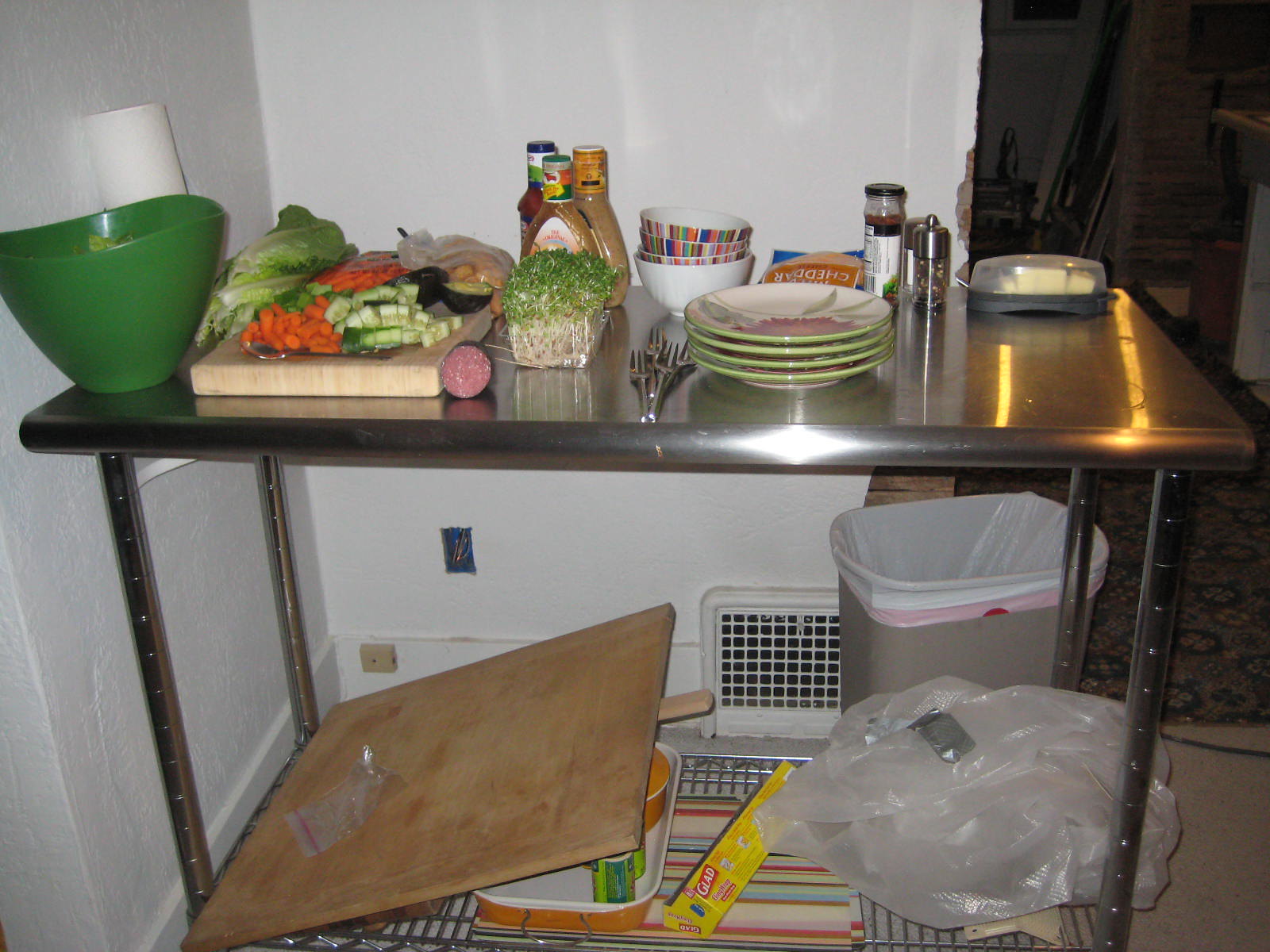An indoor scene, seemingly set in a cozy kitchen or dining area of a home. The background reveals the corner of intersecting white walls, with a door leading to another room where a carpet or rug and some indistinct chairs are visible. The adjoining room has wooden paneling and possibly a small window, although details are partly obscured. The main area has a light-colored linoleum or vinyl floor, offering a clean and neutral surface.

At the center of the image stands a metal cart, likely stainless steel, with sturdy metal legs and a grated shelf at the bottom. The shelf holds a rectangular baking dish, a large wooden cutting board, a roll of plastic wrap, and some wadded-up plastic.

Behind the cart, a gray trash can with a bag inside is noticeable. The cart's top surface is bustling with culinary activity, featuring a tall green bowl, a cutting board crowded with cut vegetables including cucumber, carrot, lettuce, and an avocado. Slices of salami, three bottles of salad dressing, three or four bowls, four plates, a block of cheddar cheese, and a salt and pepper set sit neatly arranged. Utensils and a butter dish with butter also occupy the cart, ready for meal preparation.